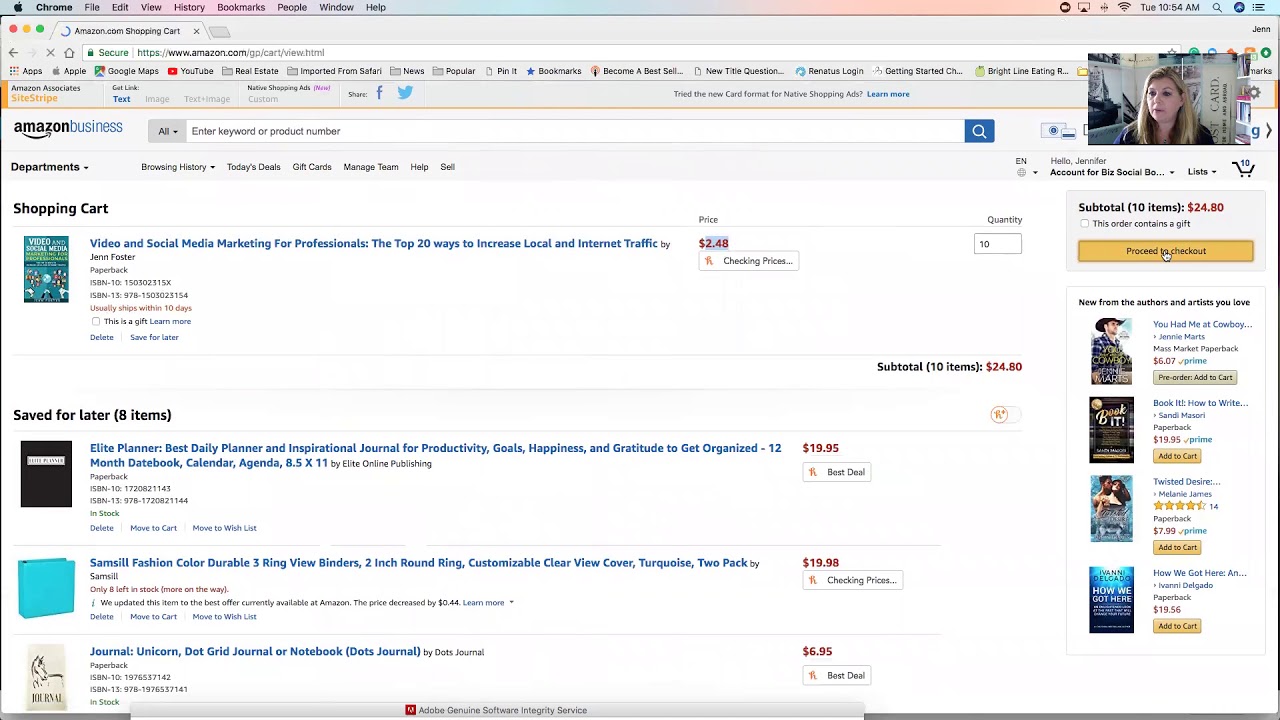The image depicts an Amazon Business home screen, showcasing various elements of the user interface. At the top, there's a blue "All" button followed by a long search bar with a microphone icon available for voice search. To the right of the search bar, a shopping cart icon is visible, along with a thumbnail image, possibly representing a book category. Below this, in blue text, is a title: "Video with Social Media: Marketing for Professionals – The Top 20 Ways to Increase Local and Internet Traffic," accompanied by additional descriptive information underneath. 

A visible quantity box indicates '10'. In the top right corner, there is a profile picture of a white female with blonde hair, drifting over her shoulders, looking sideways. Below this profile picture, the screen displays a subtotal for the cart: "10 items, $24.80," with a highlighted "Proceed to Checkout" button. Adjacent to this, a "Save for Later" section lists eight items, including a planner with a small fashion color and a journal. The mouse icon is placed over the "Proceed to Checkout" button, indicating user action.